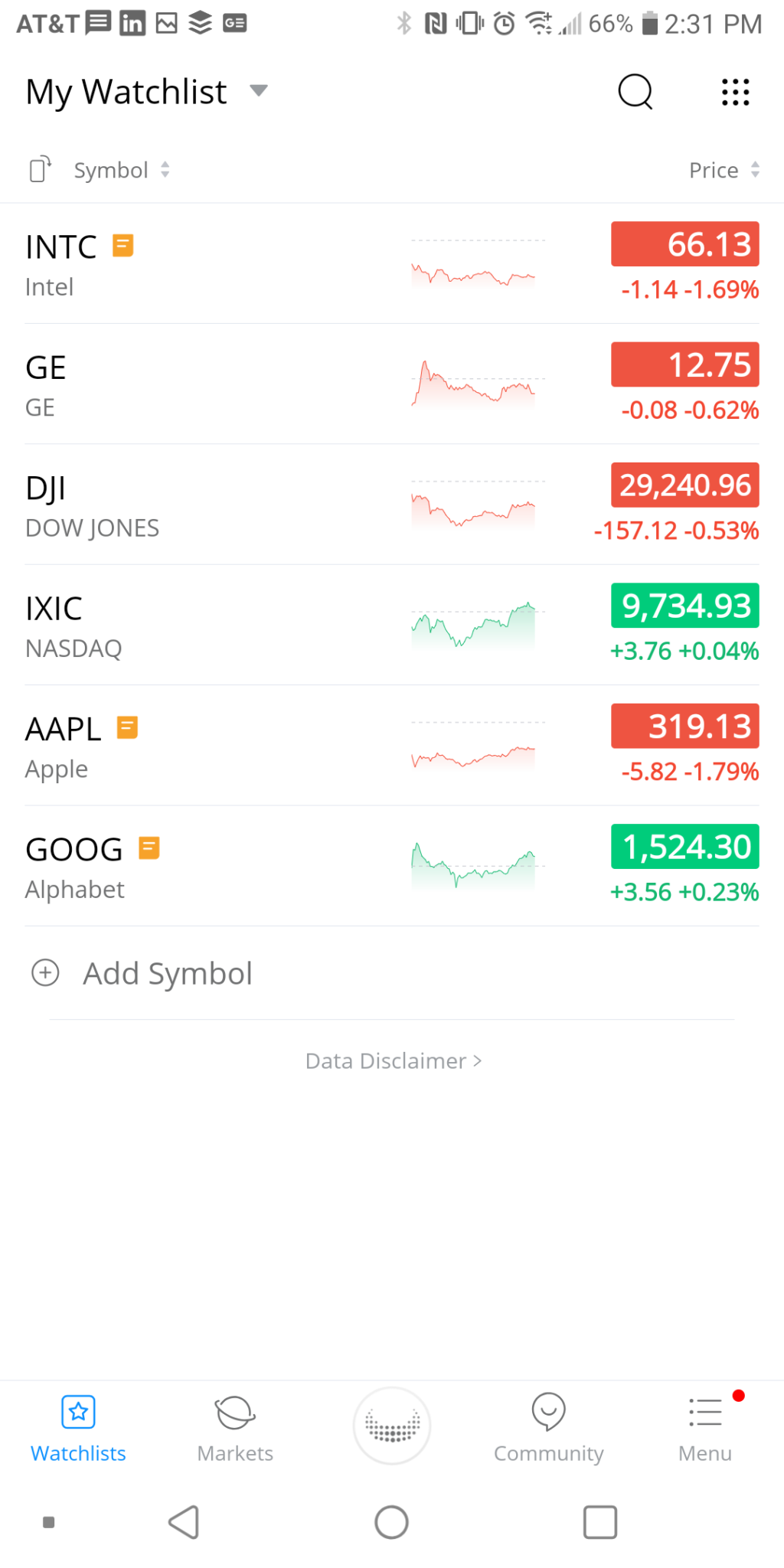The image depicts a screen capture of a mobile device interface. In the upper left corner, it displays "AT&T" indicating the phone company. Adjacent to it, the battery icon shows a 66% charge, and the current time is 2:31 p.m.

Below this status bar, to the left, the heading "My Watch List" is displayed, accompanied by a downward-pointing arrow. Under this heading, a list of company abbreviations and their corresponding names is presented:

1. **INTC** with "Intel" below it.
2. **GE** with "GE" below it.
3. **DJI** with "Dow Jones" below it.
4. **IXIC** with "NASDAQ" below it.
5. **AAPL** with an orange dot next to it and "Apple" below it.
6. **GOOG** with "Alphabet" below it.

To the right, under the subcategory titled "Price," there is a series of color-coded squares indicating the prices:

- Three sequential orange squares, each containing different numerical values.
- A green square displaying the value 9734.93.
- An orange square with the number 319.13.
- Finally, a green square showing the value 1524.30.